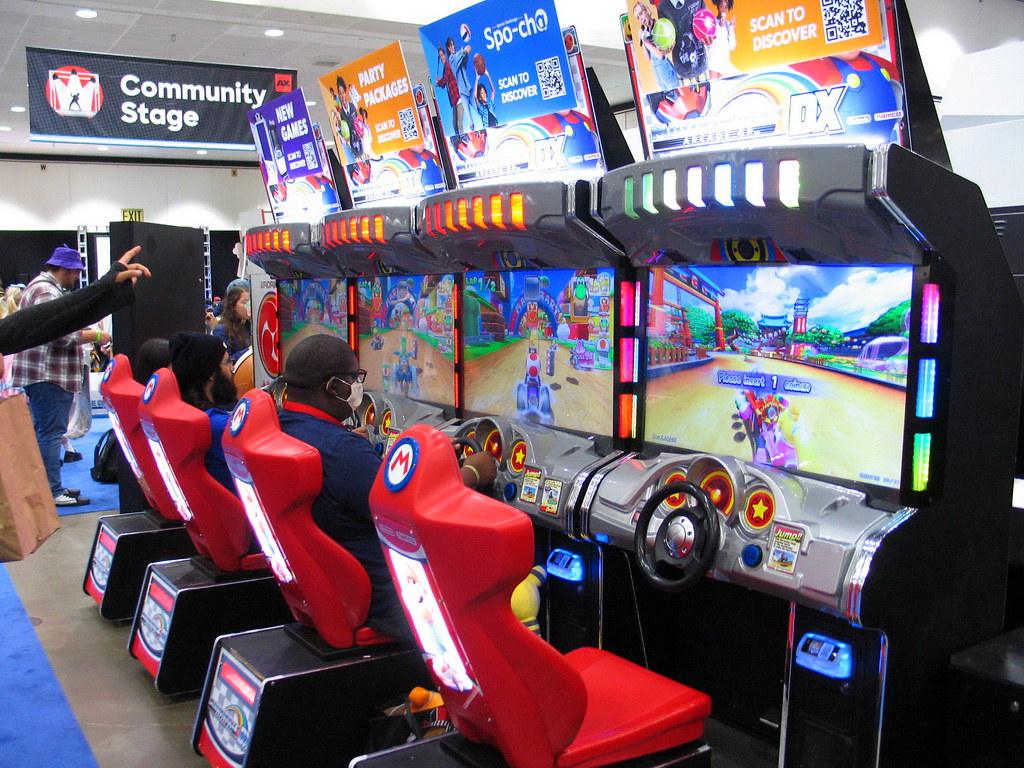In a vibrant photo captured at what appears to be a video game expo or an arcade, the main focus is on a row of four driving video game consoles prominently featuring race car seats and steering wheels. Two men are engrossed in the game, each seated in one of the distinct red chairs, with the third chair from the camera being occupied by another person while the chair closest to the viewer remains empty. Above the consoles, multiple banners and signs advertise various offerings such as "Spocha," "Party Packages," "New Games," and a QR code with the message "Scan to Discover." Adding context to the scene, the background reveals a white wall adorned with an "Exit" sign and a prominent banner labeled "Community Stage," emphasizing the lively and engaging environment of the gaming area.